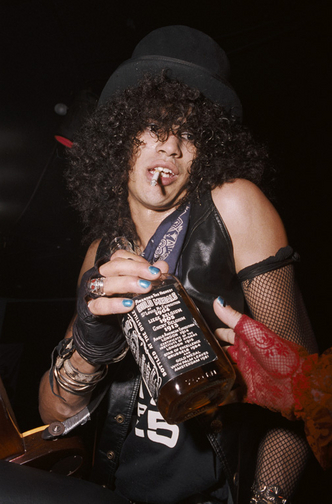The photograph captures a young Slash, the iconic guitarist from Guns N' Roses, likely during the early to mid-80s in Los Angeles. He is immediately recognizable with his signature top hat and voluminous curly hair cascading out from beneath it. Slash holds a bottle of Jack Daniel’s whiskey in his right hand, while a cigarette dangles from his slightly open mouth. He sports a black, sleeveless leather vest over a black t-shirt that features indistinct white lettering, and a black bandana wrapped around his neck. His fingers are painted blue and adorned with a red fishnet glove on his left hand. In the image, a woman with a red gauzy glove, decorated with black nail polish and visible black fingertips, is seen handing him the whiskey bottle. The background is dark, ensuring all focus remains on Slash and his party-ready appearance.